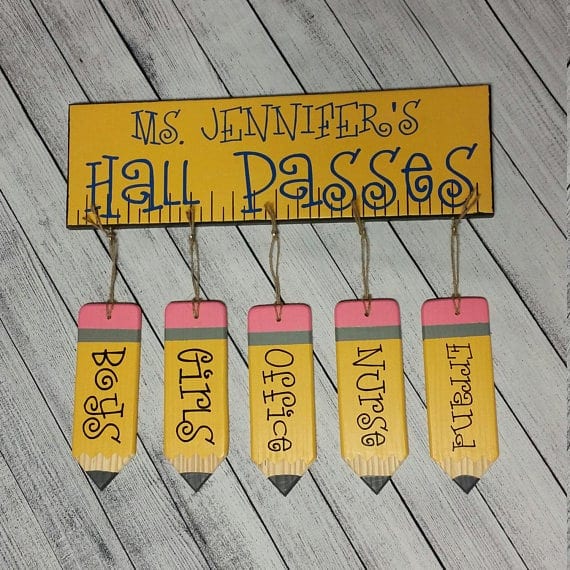The square image portrays a classroom-themed sign set against a background of diagonally aligned, sketch-like wooden boards, colored in a pale, driftwood gray tone. The focal point of the image is a horizontal yellow rectangle resembling a ruler, complete with black borders and ruler-like markings. At the top of the rectangle, it reads "Ms. Jennifer's Hall Passes" in swirled lettering.

Suspended from the ruler by tiny brown twine ropes are five adorable pencil-shaped hall passes. Each pass is designed to mimic a classic No. 2 pencil, complete with a pink eraser, a gray metal band, an orange body, a tan wood tip, and a charcoal-gray triangular lead point. The labels on the pencils from left to right read: Boys, Girls, Office, Nurse, and Errand.